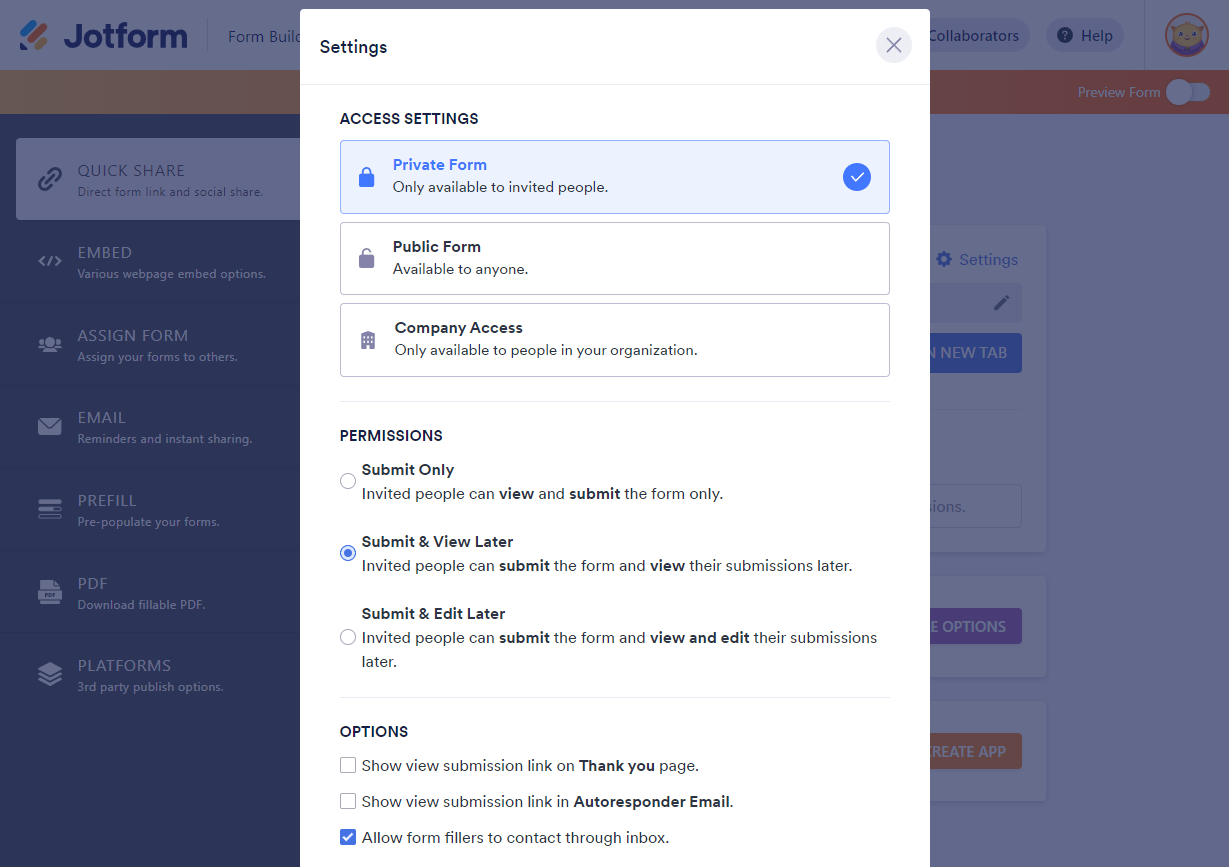A screenshot showing the JotForm interface, where the background is grayed out with a purple hue. In the upper left-hand corner, the JotForm logo is visible. The focal point of the image is a white pop-up window titled "Settings" on the left side. To the right, there's a gray circle with an 'X' inside for closing the pop-up. Below the title is a light gray horizontal line followed by the text "Access Settings."

The settings section features three options:
1. The first box includes a lock icon and reads "Private Form: Only available to invited people," with a blue circle and a white checkmark indicating it is selected.
2. The second box, outlined in gray with a white center, shows an open lock icon and reads "Public Form: Available to anyone."
3. The third box displays a building icon with six windows and specifies "Company Access: Only available to people in your organization."

Below these options, in bold, all caps, it says "PERMISSIONS," indicating different permission settings:
1. "Submit Only," marked by an open circle, meaning invited people can view and submit to the form only.
2. "Submit and View Later," indicated by a blue circle with a blue dot (selected), stating that invited people can submit the form and view it later.